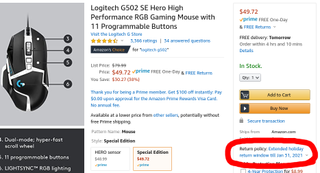This detailed caption describes an Amazon listing for a Logitech G502SE Hero High Performance RGB Gaming Mouse. The listing screenshot features an image of the mouse on the left side, set against a gray background. The mouse's key features are labeled with numbers, accompanied by white descriptive text on a dark gray background. The product title, "Logitech G502SE Hero High Performance RGB Gaming Mouse with 11 Programmable Buttons," is clearly displayed, along with the price of $49.72. 

On the right side of the listing, there are prominent buttons for "Add to Cart" and "Buy Now." Below these buttons, a refund policy is highlighted in blue text, stating, "Extended Holiday Return Window till January 31, 2021," encircled in bold red for emphasis. Additional promotional text thanks Prime members and offers a discount: "Thank you for being a Prime member. Get $100 off instantly." The listing also includes different selection options, specifically focusing on the "Hero Sensor" and "Special Edition," with the latter being chosen in this screenshot.